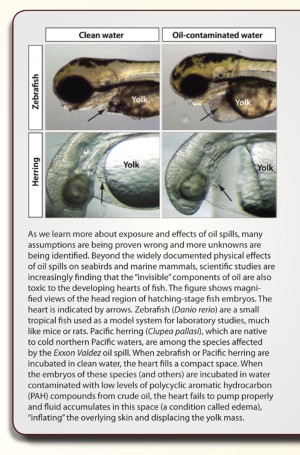A screenshot of a scanned document displays a research page examining the effects of oil contamination on aquatic life. The top section features four vibrant, color photographs comparing two species of fish, a zebrafish and a herring, under contrasting conditions: clean water and oil-polluted water. Each pair of images highlights the stark difference in appearance and health between the fish in the two environments. Beneath the photographs, a substantial text block provides an in-depth analysis discussing the detrimental impacts of oil spills on these species, emphasizing the broader ecological consequences for aquatic ecosystems.